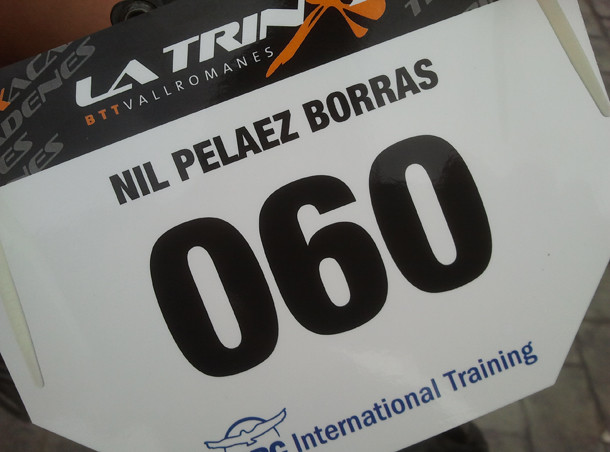This photograph captures a race bib placed on a gray brick pathway, likely signifying participation in a marathon or long-distance running event. The bib, taken from an angled perspective, showcases intricate design details: up top, a black bar inscribed with "LA TRIN BTT Valor Romanis" in both white and orange font. Below this bar, bold black letters spell out "Nil Peles Boras" with the participant number "060" prominently displayed underneath. At the bottom of the bib, "International Training" appears in purple font, accompanied by a logo to the left depicting the outline of a bird within a semicircle and the letters "RC." The whole scene is devoid of people or trees, emphasizing the lone bib on the brick pathway.